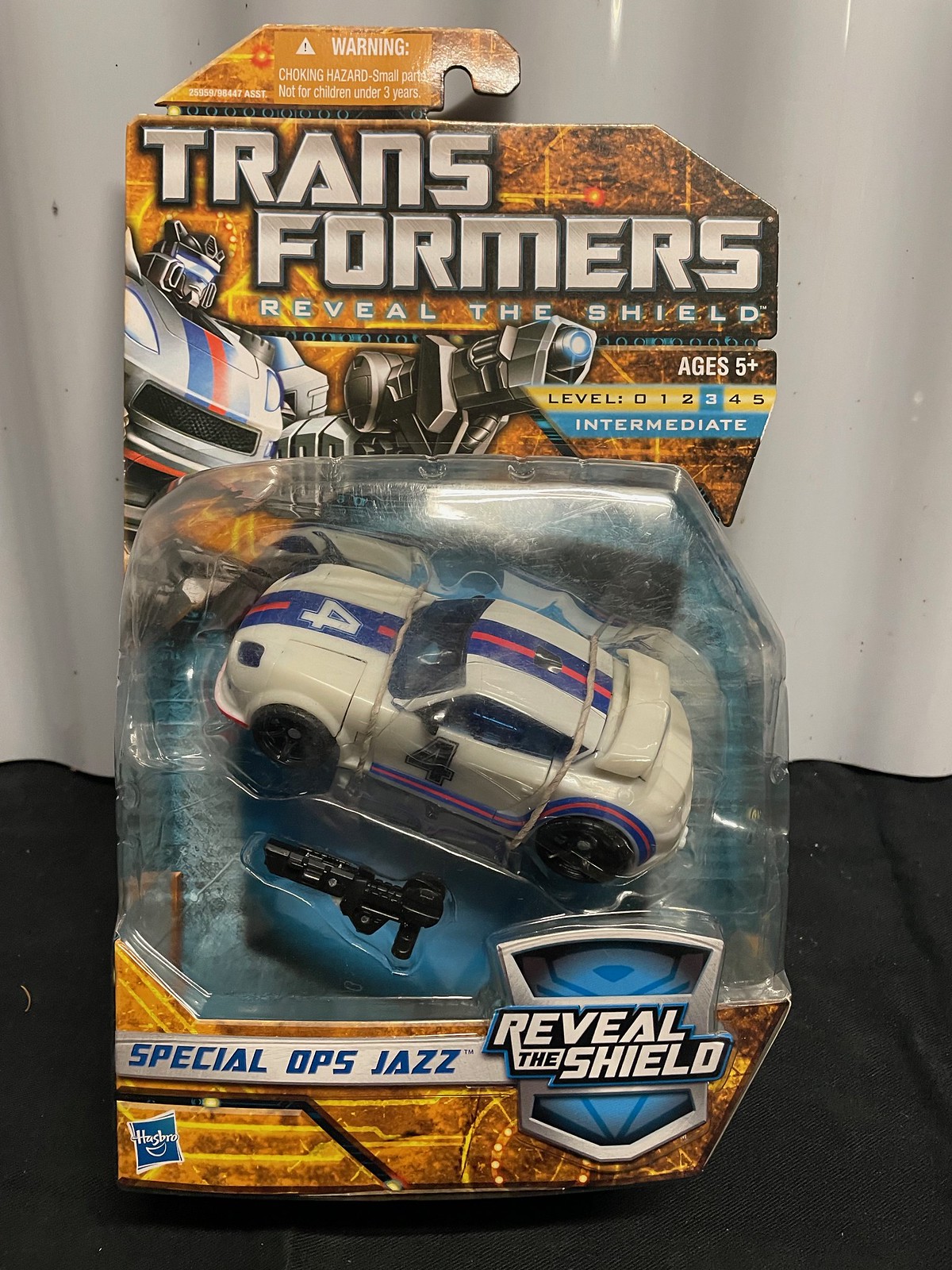The image is a color photograph featuring a toy package placed against a white background on a black surface. The package contains a toy car from the "Transformers Reveal the Shield" series. The packaging prominently displays the text "Transformers Reveal the Shield" along with a warning label at the top that reads, "Warning, choking hazard, small parts, not for children under 3." The toy, suitable for ages 5 and up, is classified as Level 3, Intermediate. The car itself is white with a blue stripe flanked by a smaller red stripe, and features a white number 4 on it. Additionally, there appears to be a small black accessory, likely a gun, included inside the package. The bottom section of the package includes the text "Special Ops Jazz Reveal the Shield," and a small Hasbro logo is visible in the bottom left corner.